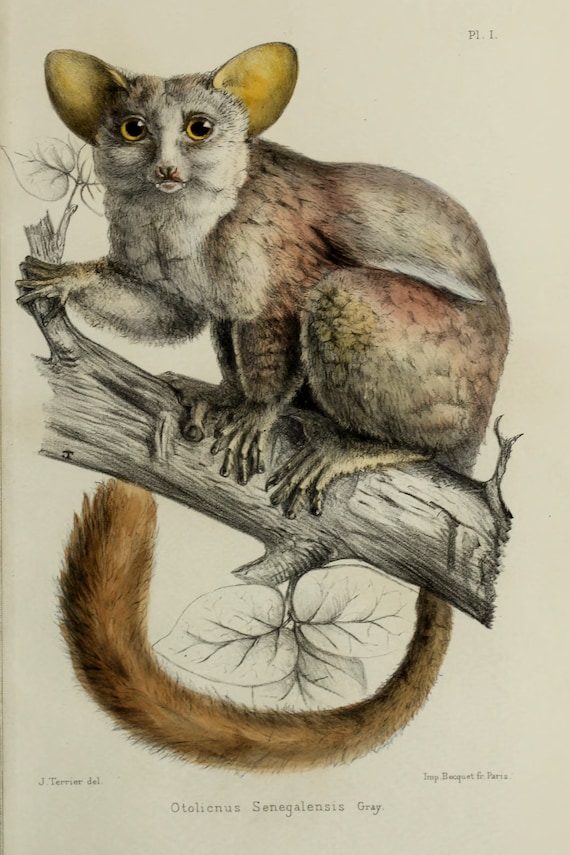The image is a detailed and colorful illustration of what appears to be a mammalian creature, possibly a lemur or marsupial, identified by the Latin name "Otiolinus senegalensis gray" displayed in small black text at the bottom. This vertically rectangular artwork features a creature with distinctive big yellow eyes and large yellow-tinted ears. The fur is predominantly gray with subtle reddish and greenish highlights, and the creature's bushy tail is brown. The animal, which has a prehensile tail and an opposable thumb, is depicted gripping a thick tree branch with three of its limbs while extending one leg to hold a side branch. The background is a grayish tone, and the lower left and right corners include the artist's name, noted as J. Terrier, and a reference to Paris. The illustration suggests an air of antiquity, possibly due to the off-white color of the aged paper.